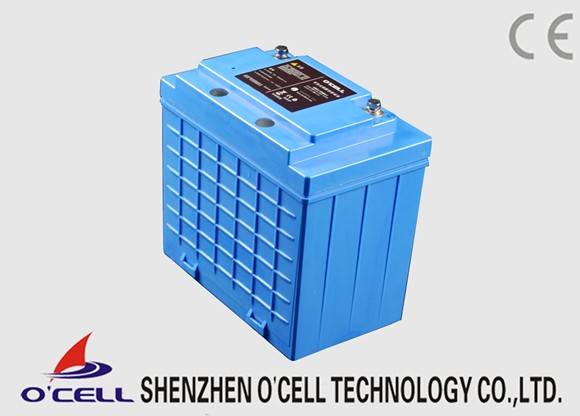The promotional image features an industrial component prominently displayed against a light gray background. At the center of the image is a rectangular blue box with distinctive ridges along its sides and vertical lines running down. The box likely represents a battery or a fuel cell, as suggested by its design and structure. Towards the top of the blue box, there is a black label with white text, flanked by two silver nubs that appear to serve as terminals. In the top right corner of the image, gray text reads "CE," denoting compliance with European safety standards.

In the bottom left corner is the brand logo featuring a red, triangular cell-shaped tank with two curved blue lines extending from it, alongside blue text that reads "Ocell." The bottom of the image bears the manufacturer’s name in black text: "Shenzhen Ocell Technology Company Limited." This detailed layout highlights the company's branding and the industrial nature of the component being advertised.